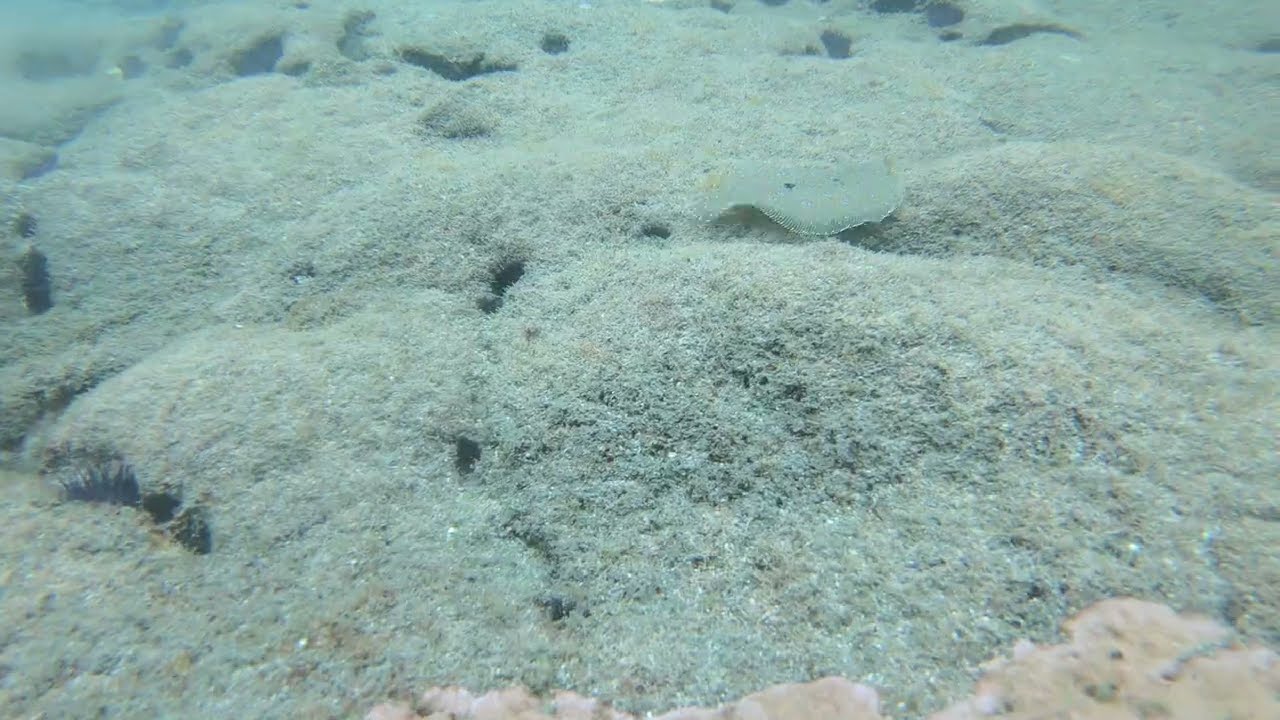The image is an extremely close-up shot revealing a landscape-like scene heavily influenced by natural elements. The central focus is a piece of land covered in green, hairy mosses, interspersed with dark green or black holes. Amidst this lush area, there is a prominent round green leaf. Towards the bottom right, the texture transitions into a light brown area. Adding to the complexity, parts of this scene appear to mimic underwater sand, transitioning from yellowish to blue, with sparkly textures. Embedded in this blue sand is a small, flat stingray, blue with white spots, blending seamlessly with its surroundings. Scattered giant rocks add another layer of detail, while the stingray itself appears isolated without companions. The composition further evokes the image of a fluffy, white substance like cotton or snow, with ridges and open blemishes, enhancing the textured, multi-faceted appearance of the scene.